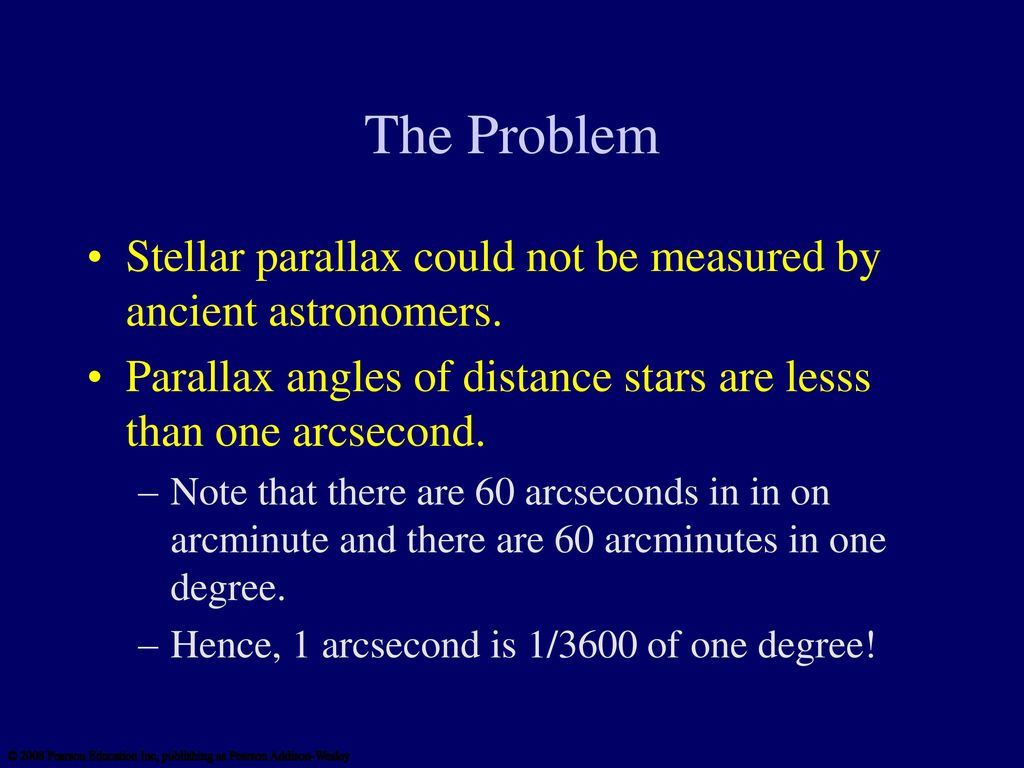The image, resembling an excerpt from a PowerPoint slide, features a dark blue background with a central heading in white letters titled "The Problem." Beneath this heading are two primary bullet points in yellow text: "Stellar parallax could not be measured by ancient astronomers," and "Parallax angles of distant stars are less than one arc second." Below these points, in white text, are two notes: "Note that there are 60 arc seconds in one arc minute and there are 60 arc minutes in one degree," and "Hence, one arc second is 1/3600th of one degree." Additionally, the bottom left corner contains blurred black text that partially reads "copyright," making it difficult to decipher the complete message.